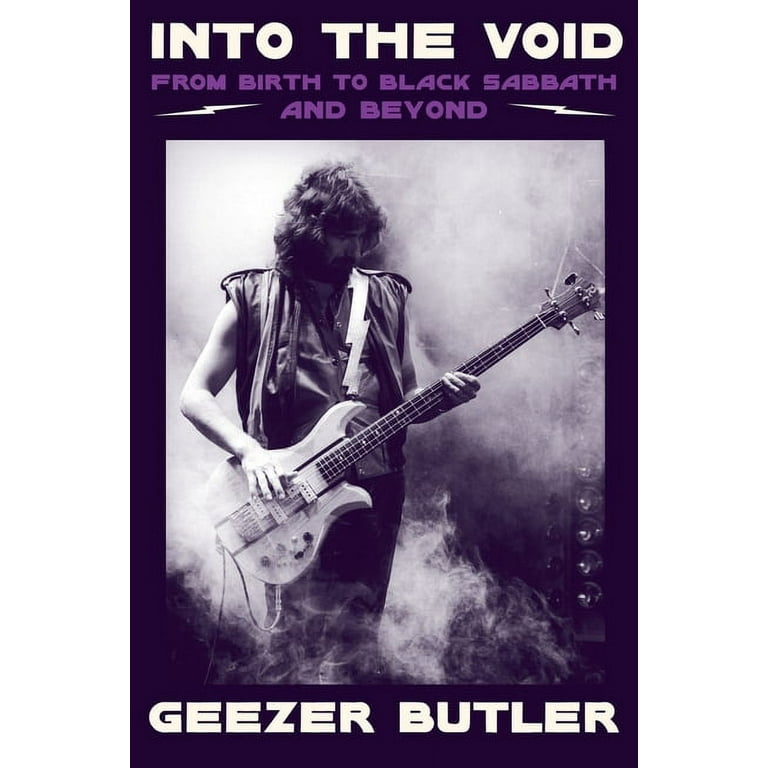The poster titled "Into the Void: From Birth to Black Sabbath and Beyond" features a monochromatic, moody image at its center, capturing a guitarist deeply immersed in his music. Surrounded by swirling smoke from a stage machine, the man with long brown hair, a mustache, and a beard, is clad in dark clothing accented by a zigzag, lightning-like guitar strap. Stage lights subtly illuminate the scene from the background. The musician, identified as Geezer Butler, is depicted playing an electric guitar while intently focusing on his finger placement. The poster's dark tones are contrasted by some white and light purple text, adding to its intense, rock star aesthetic.